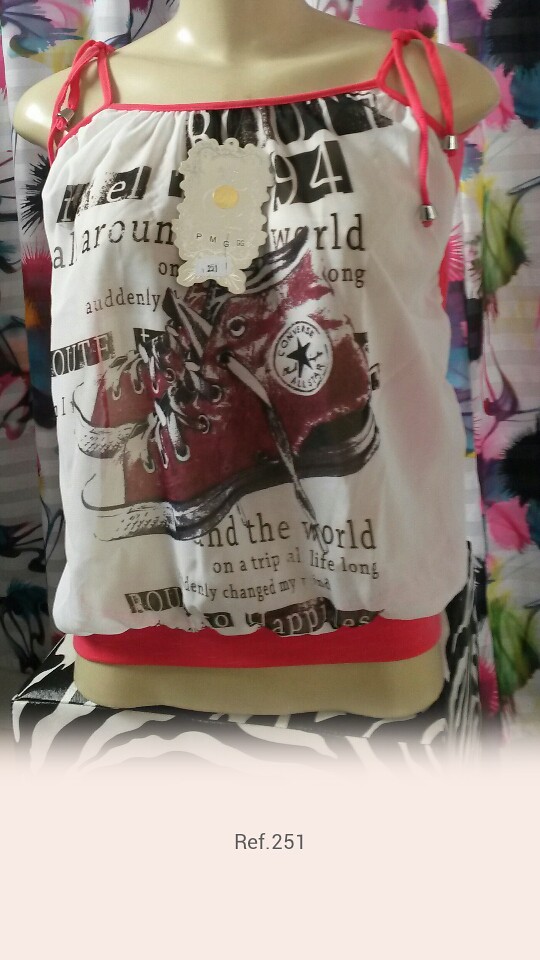This photograph captures the torso of a female armless mannequin dressed in a sleeveless white tank top with pink shoulder straps tied into bows. The tank top features an illustration of a pair of red Converse All-Star sneakers with white laces and soles. Surrounding the shoes is black text that partially reads, "Around the world, On a trip, Lifelong, Suddenly changed." The mannequin is seated on a zebra-print display cube. A tag or label saying 'PMG' is pinned to the tank top, and below the image, the text "Ref.251" is clearly visible. Curtains can be seen in the background, adding to the scene's context.